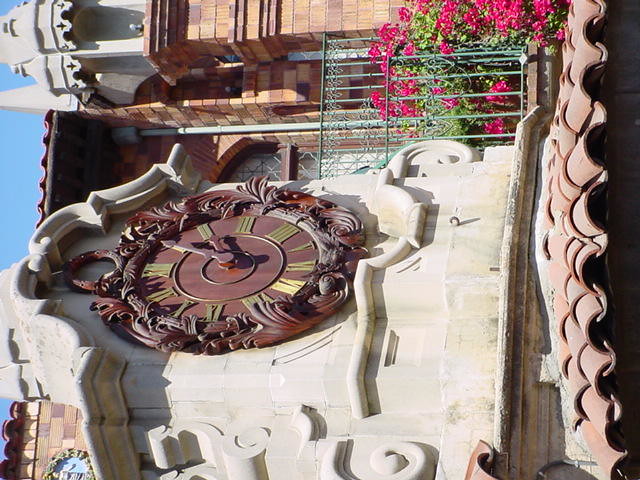The photograph, which is oriented sideways, captures an ornate outdoor clock that appears to be part of a larger architectural structure. The clock is a rich brown color, featuring gold Roman numerals and intricate detailing. It shows the time as approximately 2:08. The backdrop includes a grand structure with detailed engravings resembling crown molding at the top and a curling line at the bottom. Below and behind the clock, the scene transitions into a variety of textures and colors: 

- To the left, there's a massive building adorned with comprehensive designs resembling a mix of brick and light gray stone.
- To the right, a gray or green fence surrounds a balcony, behind which vibrant pink flowers with green leaves are visible.
- A section of a swirly roof can be seen at the bottom of the sideways photograph, next to a clay or stone background.

All these elements combine to create a vivid, detailed image that would be complete if rotated 90 degrees to the right.